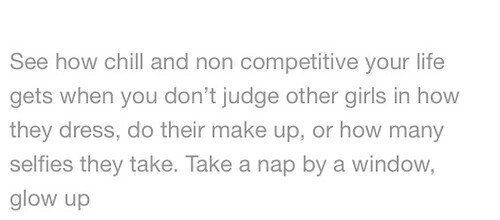The image features five lines of light blue text against a plain white background, presented in a modern casual font. The text reads: "See how chill and non-competitive your life gets when you don't judge other girls in how they dress, do their makeup, or how many selfies they take. Take a nap by a window, glow up." The lines are straightforward and unindented, with each phrase formatted for clarity and impact. The overall message is inspirational, encouraging kindness and self-improvement, without any additional images or decorative elements.